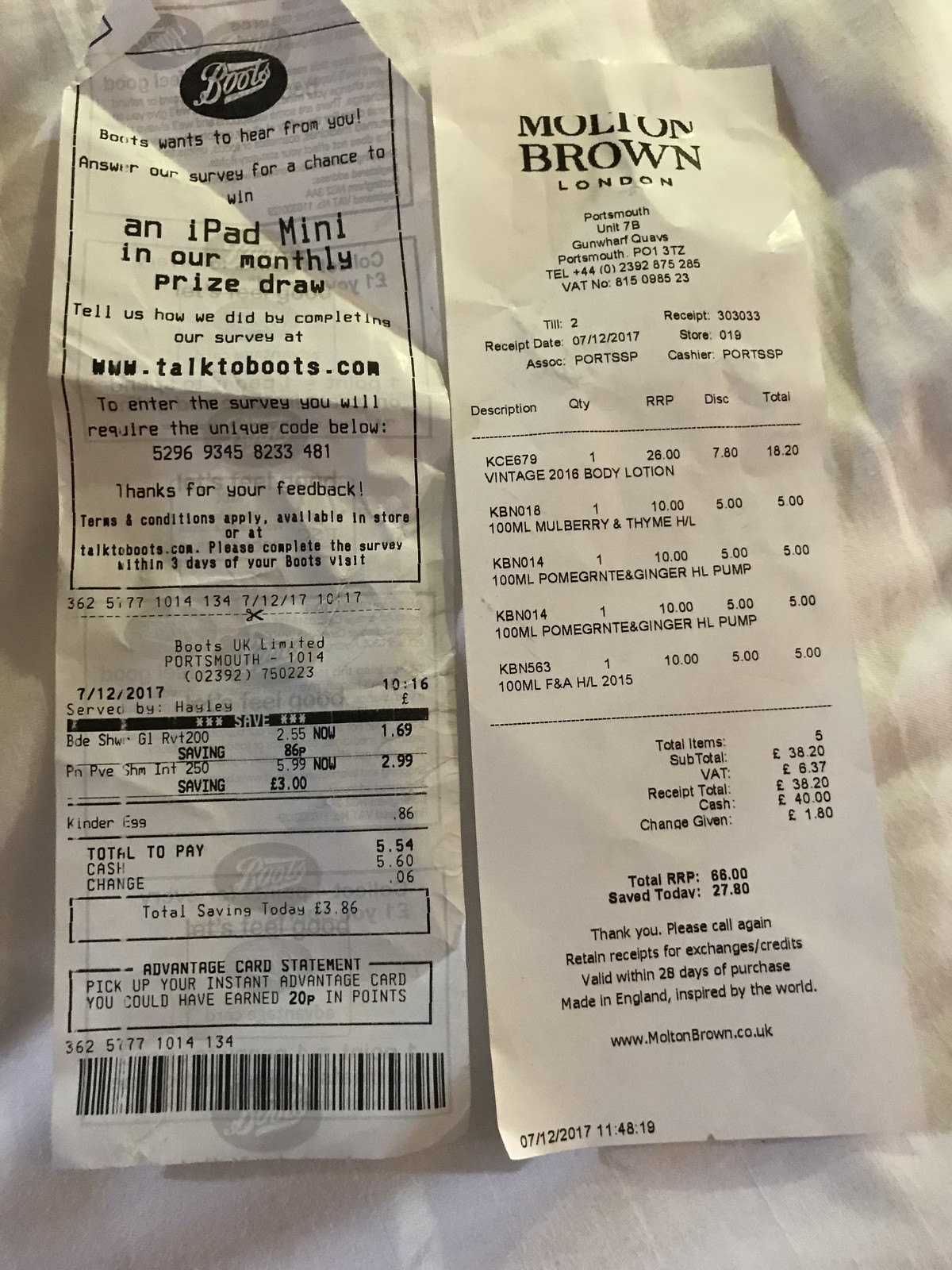In this photograph, we see two receipts lying on a white paper surface, which is placed over a table draped with a white tablecloth. One receipt is from Boots, and the other is from Molton Brown London, indicating recent purchases from these two stores. Both stores are located in Portsmouth, United Kingdom, as deduced from the addresses visible on the receipts. The Boots receipt highlights a special promotion, offering a chance to join a sweepstakes for an iPad mini and a monthly draw upon completing a survey. The total expenditure at Boots is £5.60. Meanwhile, the amount spent at Molton Brown London is noted as £38.20.